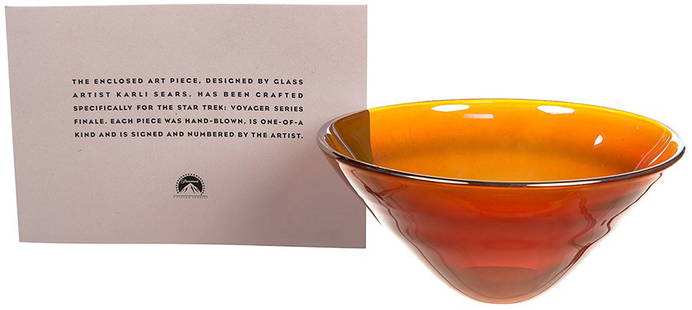The photograph showcases a uniquely designed amber glass bowl and an accompanying informational card, all set against a pristine white backdrop. The bowl, positioned on the right side of the image, features a narrow base that gently slants outward, culminating in a wide, open mouth. Its translucent amber hue allows light to pass through, highlighting the craftsmanship. To the left, a light gray card with black type details the provenance of the art piece: "The enclosed art piece, designed by glass artist Carly Sears, has been crafted specifically for the Star Trek Voyager series finale. Each piece was hand-blown, is one-of-a-kind, and is signed and numbered by the artist." At the bottom of the card, the Paramount Studios logo is prominently displayed, attesting to its official endorsement.